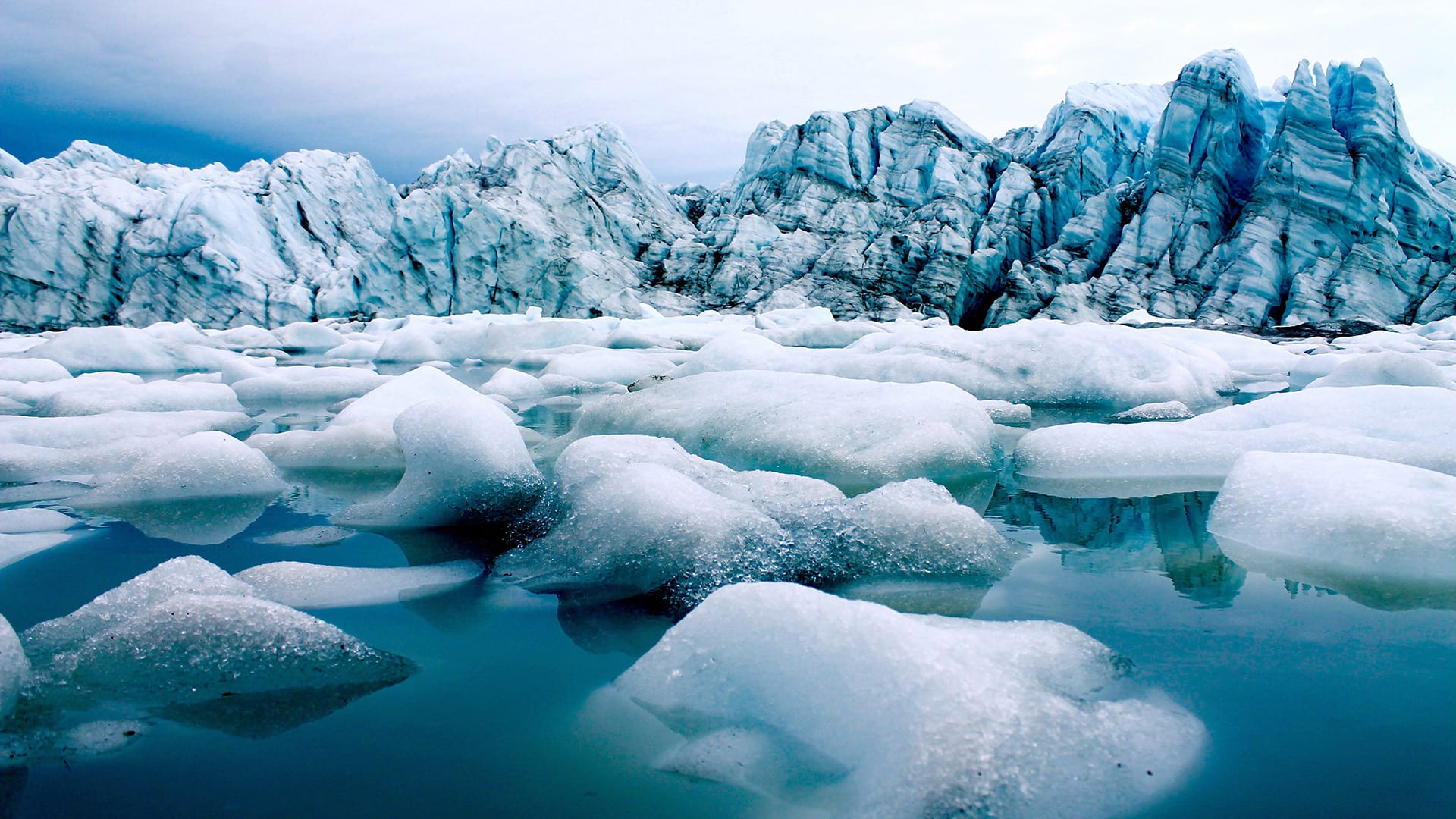This photograph captures a striking polar landscape. The background features a mostly white sky, with a deeper blue visible towards the upper left. Just below the sky, rugged mountains span the horizon; their surfaces show a mix of potential snow cover and exposed rock, adding texture with visible lines, cracks, and creases. The mountains, particularly on the left, exhibit hues ranging from light to dark gray. In the foreground, the scene transitions to a landscape dominated by pure white ice and snow, undisturbed and clean. The ice forms small mounds and peaks, interspersed with patches of dark blue, slightly green-tinted water, indicating areas where the ice is melting. Some parts of the water reflect the textured, blue and white mountains. The ice remains prominently above the water, creating a vivid contrast that emphasizes the pristine and harsh beauty of this arctic environment.